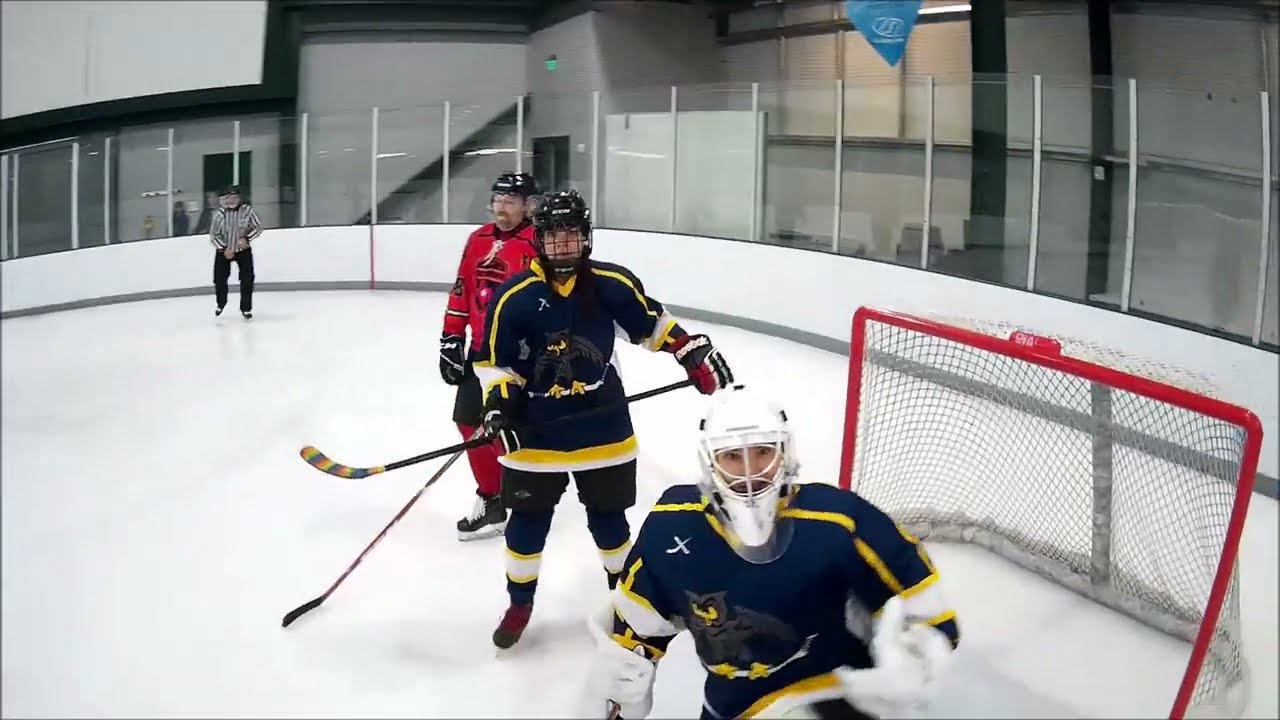The photograph captures a detailed scene of an indoor ice hockey rink mid-game. The ice rink is predominantly white with a white border and features a glass partition with vertical metal spines dividing the glass into sections, providing a clear view beyond the rink. Central to the image are three hockey players positioned near a red-trimmed goal with a gray net. The first player, clad in a red jersey, red pants, and a black helmet, stands towards the left. The middle player dons a black helmet, a black jersey with yellow and white accents, black pants, and matching yellow and white socks. The player closest to the camera is equipped with a white helmet and a black jersey featuring yellow and white details. To the left in the background, a referee dressed in black and white stands distant from the main scene. The overall composition highlights the action within the rink, with the players and referee enhancing the sense of an ongoing hockey game.